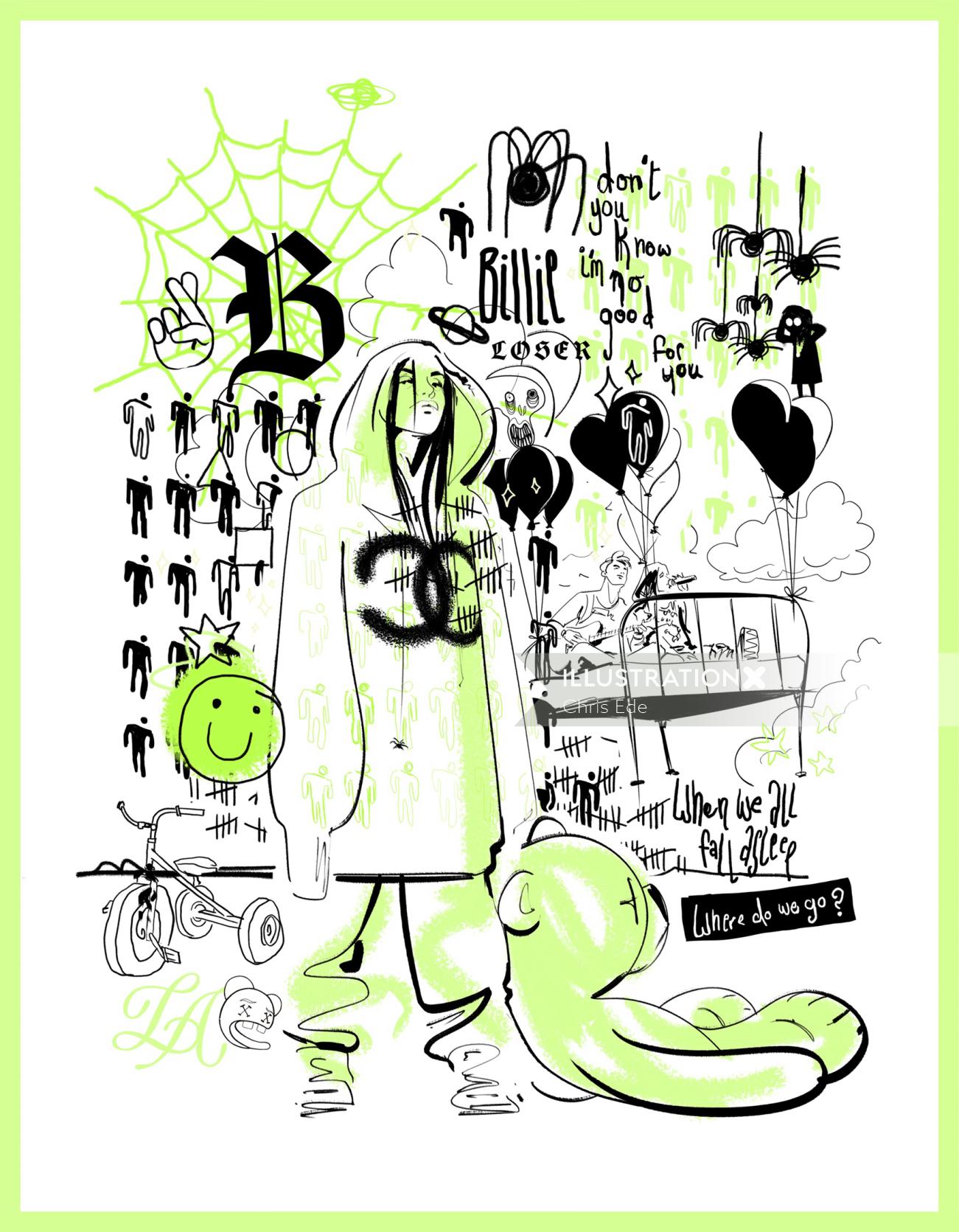The image features a detailed drawing rendered in black, white, and lime green tones. At its center stands a person with long black hair, wearing an oversized, hooded white sweatshirt adorned with a distinctive logo: two overlapping C's, one backward, creating an oval shape amidst a pattern of tally marks. The character, possibly a young man, wears baggy pants and a scowling expression. They clutch a large, lumpy lime green teddy bear leaning against their leg, and next to this, on their left, is a sketch of a tricycle. Floating near the teddy bear, above it, is a lime green smiley face reminiscent of a Walmart logo, while to its left are black-and-white silhouette icons of people arranged alternately. A black spider dangles in front of the person, contributing to the overall sense of strangeness. The upper left corner displays a light green spider web with a black letter 'B' trapped in it, and various spiders hang throughout the image. There's also a whimsical scene of someone on a bed playing a guitar, with black balloons tied to the bed's rails. The image is sprinkled with text including "don't you know I'm no good for you" and "Billy loser" at the top, and "where do we go" at the bottom right encapsulated in a black box with white text.